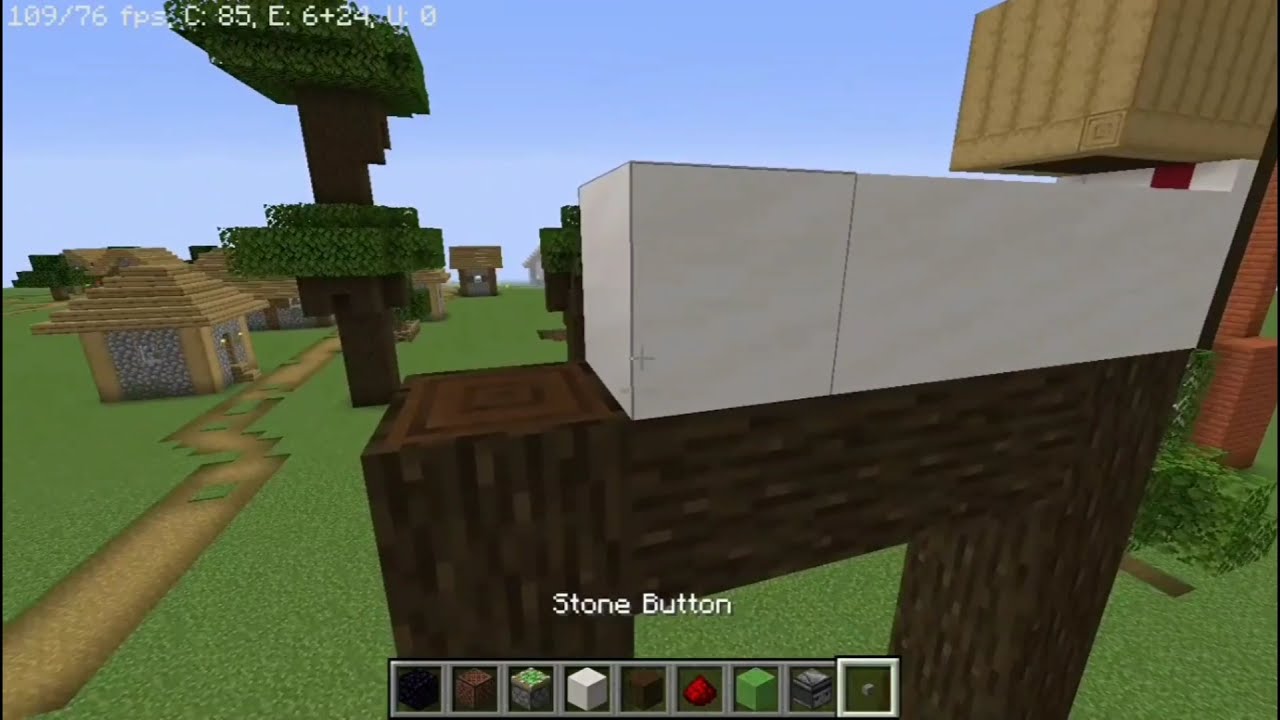The image appears to be a high-definition screenshot from the video game Minecraft, showcasing a bright, clear daytime with a blue sky and some scattered clouds. In the upper left corner, white text reads "109-76 FPS," followed by additional game data like "c85 e6 + 24 u0." The scene features a green field on the left, home to a small building with a gray, stone-like exterior and a brown, stacked roof that narrows towards the top. Adjacent to the building is a narrow brown pathway that starts at the lower left corner of the image and winds upward, eventually curving to the left. Flanking this path is a large tree with a thick brown trunk and lush green foliage. In the foreground, there is a brown archway constructed from blocks, topped with some white elements. Towards the bottom of the image, the text "Stone Button" is visible in white, and below it are icons of different gray squares with various objects inside, presumably for selection and placement in the game.